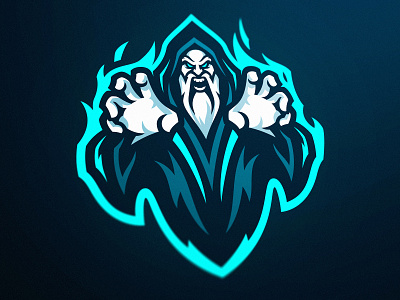The image is a graphic design featuring an elderly wizard with a ghostly appearance. He is dressed in a robe that combines dark blue, light blue, and teal hues, and wears a hood that partially obscures his bald head. The wizard has striking white facial hair, including long, well-defined eyebrows, a mustache, and a flowing beard. His piercing ice-blue eyes and bared teeth give him an angry expression as he stares directly at the viewer. Both of his wide, white hands are outstretched, fingers extended as if he's about to grasp something, surrounded by jagged teal flames that extend from his hands to the sides of the image. The background of the design transitions from a more blue-black shade to a lighter navy blue toward the top right, enhancing the mystical and fiery aura surrounding the wizard.